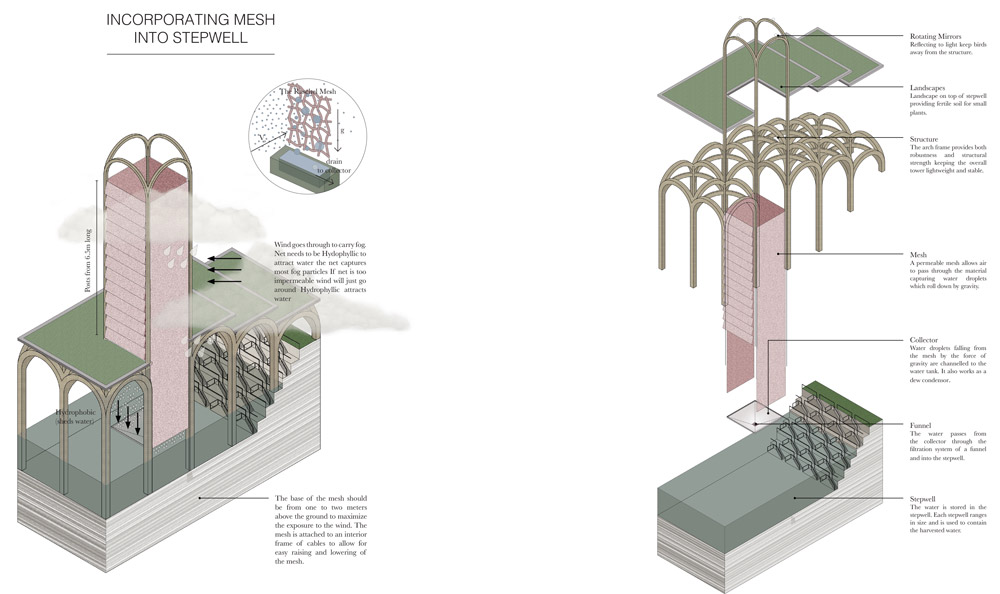This detailed technical illustration demonstrates the incorporation of mesh into a stepwell structure, emphasizing its architectural and functional components. The featured diagrams, close-ups, and schematics provide comprehensive insights into the design and installation process.

On the left side, the diagram showcases a sliced cross-section of the stepwell. It's highlighted by different colors, such as green representing the landscaped top and a pink-hued mesh. The stepwell assembly is organized to show both how it fits together and its functional internals, including integration points for the mesh.

Prominently labeled "INCORPORATING MESH INTO STEPWELL," the left section of the illustration dives into the functionality: wind flows through to carry fog, and the hydrophilic mesh captures water particles. The details specify that the mesh should be mounted 1 to 2 meters above the ground to maximize wind exposure and is attached to an internal cable frame for adjustable positioning.

The right side features segmented schematics and extensive descriptions. These explain the installation of a mesh drain, the role of rotating mirrors to deter birds, and the landscape features on top of the stepwell. Specific notes discuss the hydrophilic properties of the net, its permeability to optimize water capture, and the need for structural stability provided by an arch frame. 

Further annotations define various systems: the mesh, acting as a water collector, funnels droplets into a reservoir; the filtration system channels water into the stepwell, storing it for future use. Each stepwell's size varies, adapting to contain harvested water efficiently. The detailed text includes seven paragraphs that articulate these components and installation guidelines meticulously.